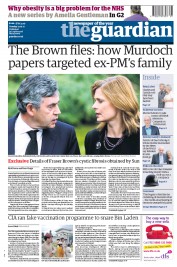In this vertical-oriented image, captured as a screenshot from The Guardian's website, the blue header spans the width of the image at the top and prominently displays "The Guardian" in large text. Beneath the header, on a white background, the text reads: "The Brown Files: How Murdoch Papers Targeted XPM's Family." 

Just below this text, there is a photograph of a man and a woman, both Caucasian and well-dressed, facing each other. Further down, there is text comprising an article, though the text and headline are too small and blurry to discern. 

Continuing to the next section, another article headline appears with a smaller image embedded within the article. Along the right-hand side of the image, several smaller images are aligned vertically. These could represent additional articles or advertisements. Notably, a red telephone is visible at the bottom of these side images.